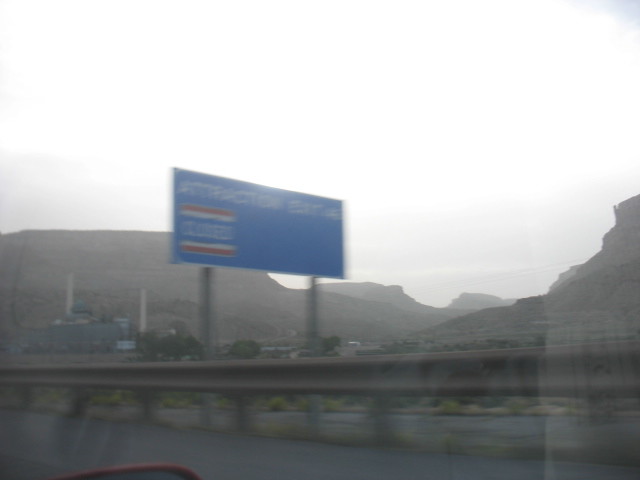A semi-blurry, hazy photograph captures an outdoor scene from inside a red car, identifiable by the visible top portion of its red side mirror. The image is taken through the car window, with a guardrail running parallel to the vehicle on the right-hand side. Beyond the guardrail, a misty, indistinct range of hills or small mountains stretches across the background beneath a hazy sky. Centrally positioned in the image is a large blue sign with white text, partially obscured by the blurry quality of the photo. Prominently displayed on the sign are red and white lines highlighting the word "CLOSED," although the exact subject of the closure remains unreadable. The overall composition reflects a moment captured in transit, amidst a scenic yet slightly obscured landscape.